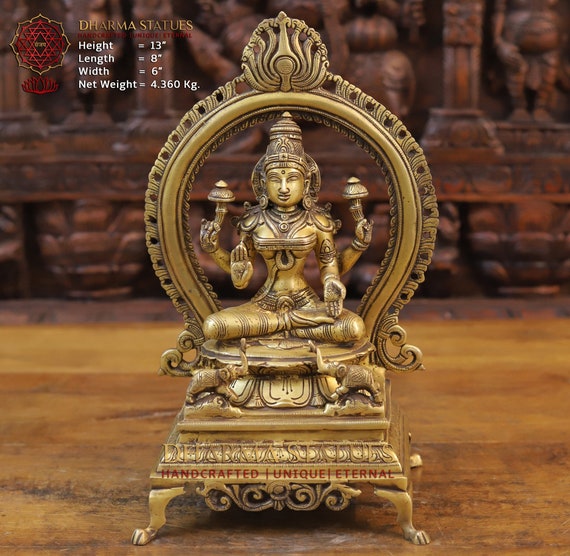The color photograph showcases a small, handcrafted, intricately carved metal statue perched on a wooden base with curved feet that resemble an ottoman. The statue depicts a deity, likely a Hindu goddess, sitting cross-legged in a meditative pose, with four arms—one hand extended palm up, another raised as if signaling to stop, and the remaining two arms positioned differently. The deity is adorned with an ornate headdress and surrounded by a detailed, horseshoe-shaped halo arch with traditional embellishments. Flanking the base of the statue are two elephants, standing on either side. The base of the statue features red text reading "Dharma Statues, handcrafted, unique, eternal." In the upper left corner of the image, white text details the dimensions and weight of the sculpture: height 13 inches, length 8 inches, width 6 inches, and net weight 4.360 kilograms. Blurred elements in the background suggest a hand-carved wooden backdrop.